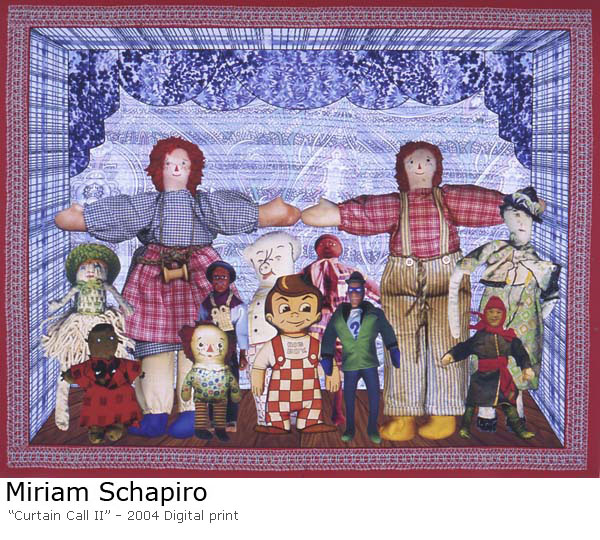The square image titled *Curtain Call 2* by Miriam Schapiro, a 2004 digital print, resembles a quilt with its intricate layout and vibrant colors. The artwork features a red border with a thicker patterned interior border of red and white. The background showcases a blue and white color scheme with interconnected half circles at the top and horizontal stripes underneath.

Centered in this whimsical setting are two prominent Raggedy Ann-style dolls, each with red hair and distinct outfits: the doll on the left wears a checked blue and white top with a red and white plaid skirt, while the doll on the right sports striped brown and white suspenders, yellow shoes, and a red and white plaid top. Their outstretched arms touch each other, creating a sense of connection.

Surrounding these main figures are approximately ten smaller dolls, dressed in various old-fashioned clothing patterns of blue, red, and seersucker stripes. Among them are additional notable characters, including a joyful pig and a boy with swooshed-up hair in red and white checkered overalls, as well as a character reminiscent of Bob's Big Boy, identifiable by his suspenders and signature look.

The entire scene appears to take place on a wooden tile floor, enclosed in a box frame with red embroidered edges. At the bottom left corner, beneath the red border, black text reads "Miriam Shapiro" followed by the title "Curtain Call 2" in smaller script.